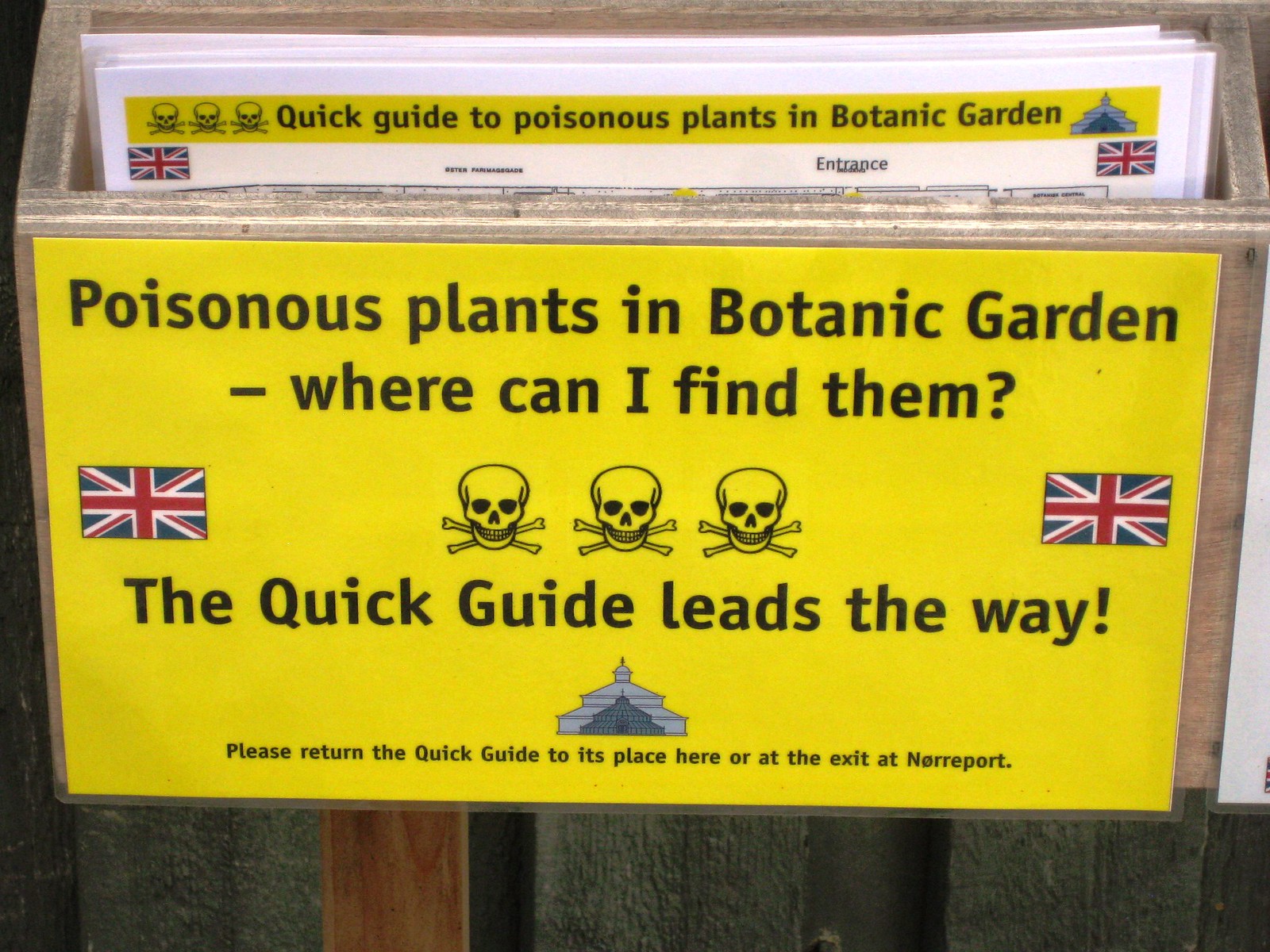The image depicts a wooden box mounted on a wall that serves as a holder for informational pamphlets about poisonous plants in the Botanical Garden. The front of the box features a prominent yellow sign with black text. At the top, the sign reads, "Poisonous Plants in Botanic Garden," followed by the question, "Where can I find them?" The design includes three central skull and crossbones illustrations flanked by small United Kingdom flags on both the left and right sides. Below the skulls, the text states, "The Quick Guide leads the way." At the bottom, there is an illustration of a small chapel-like building with the instruction, "Please return the Quick Guide to its place here or at the exit at Norport." Inside the box, several pamphlets are visible, with the top one titled "Quick Guide to Poisonous Plants in Botanic Garden." The colors of the flags are red, white, and blue, contrasting with the yellow background and black text of the sign. The entire setup suggests informative material aimed at guiding visitors through the garden while cautioning them about toxic plant species.